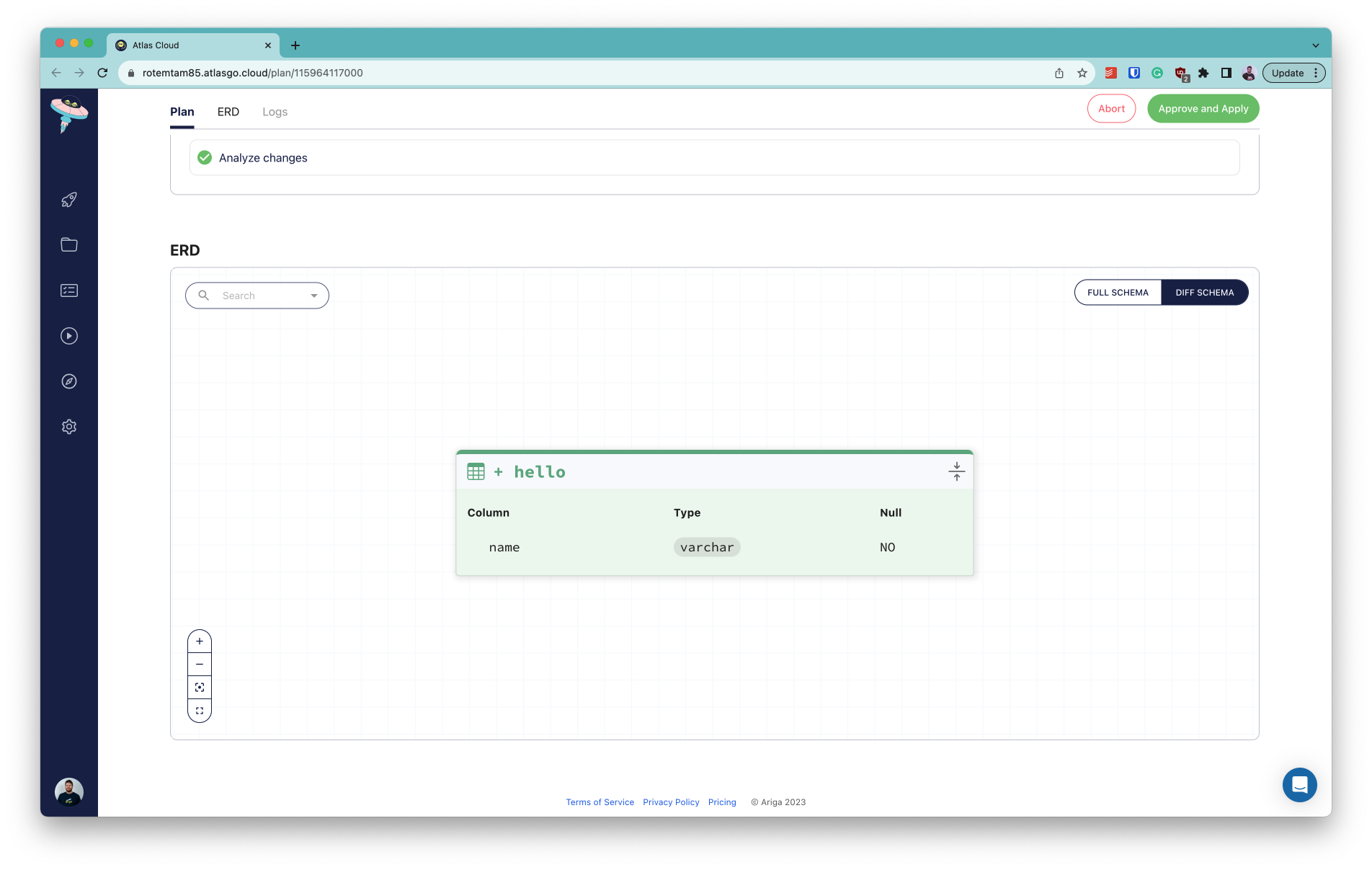This image appears to be a screenshot taken from a MacBook, as indicated by the distinct red, yellow, and green traffic light icons at the top left of the screen. Below these buttons, a UFO-like icon featuring two green aliens and a pointed or flaming base can be seen, alongside a series of additional icons: a rocket, a file folder, a play button, an unfamiliar pyramid-like symbol with a circle, and a gearbox.

At the top of the screen, a tab labeled "Atlas Cloud" is visible, with an option to close it or add a new tab. Directly beneath this tab, the text "R-O-T-M-T-A-M-85" indicates the origin of the website being viewed. The primary content area shows three tabs: "plan," "ERD," and "logs," with "logs" being grayed out, and "plan" underlined in blue, signifying it as the active tab. The "plan" section has a green check mark next to "analyze changes."

Below this, there is a larger section labeled "ERD," featuring a search function in the top left corner. To the far right, options for "full schema" and a currently selected "different schema"—highlighted in a black or blue shade—are present. Underneath the schema options, the text "calendar plus hello" appears within a green box.

The detailed view includes a table headers "Column," "Name," and "Type," the latter showing a button labeled "bar chair" and indicating that "null" is not allowed. There are also plus and minus buttons for adding or removing entries, and a maximize option. 

In the bottom right corner, a comment section is available. Just above the "analyze changes" note, there are two action buttons: "abort" in red text and "approve and apply" in green. This detailed description showcases various UI elements and tools within the viewed application interface.